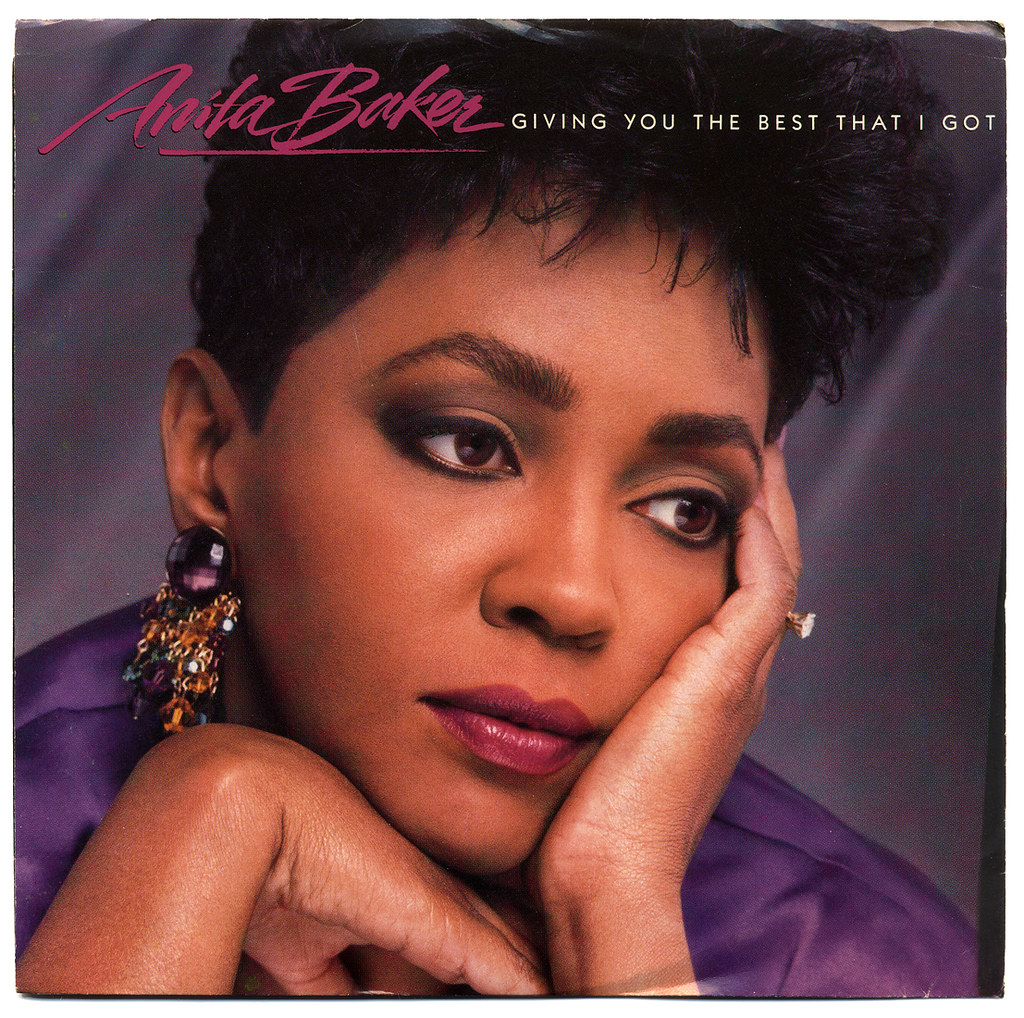This is a detailed promotional photo likely for Anita Baker's album or single, "Giving You the Best That I Got." The top of the image features her name in italic cursive, underlined by dark pink lettering, and just beside it in white text is the title, "Giving You the Best That I Got." Below the text is Anita herself, centered in the image with her face resting on her left hand and her right hand positioned under her chin. She is wearing a purple shirt paired with a striking purple earring adorned with dangly gold and light blue accents. Her look is completed with red lipstick, eye mascara, and painted eyebrows, framing her short hairstyle. Anita gazes off thoughtfully to the right, against a gray backdrop that suggests a curtain. The image, showing signs of wear such as apparent folding marks at the top, appears to be a scanned promotional record cover.